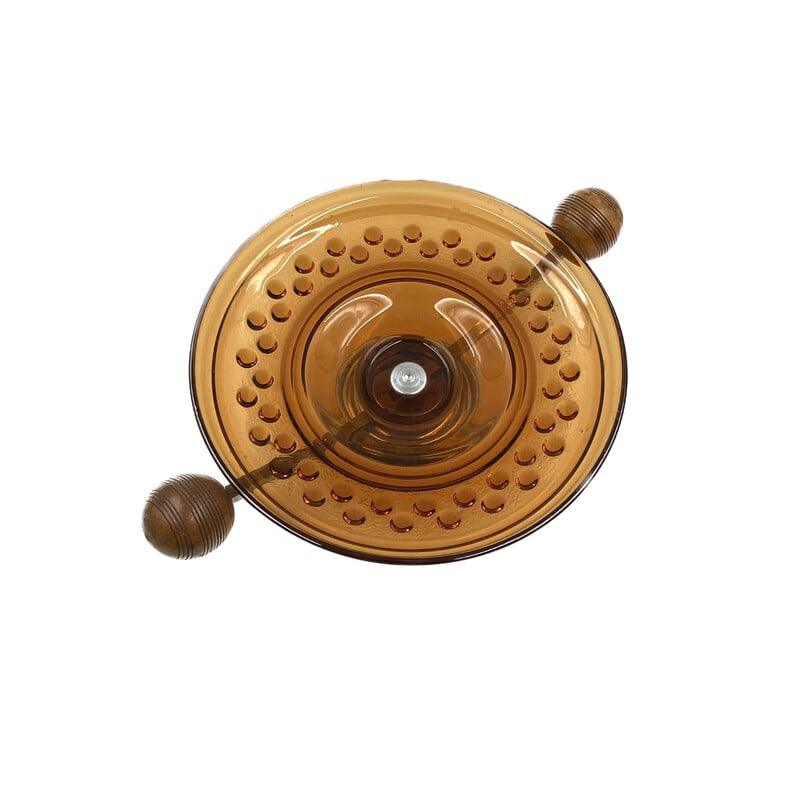The image depicts the top view of a semi-transparent, light tan, glass-like round container, possibly a bowl, against a white background. The surface of the lid is adorned with numerous bubbly, indented dots, adding a textured feel. Emerging from the center is what appears to be a wooden handle, anchored by a visible silver screw. Extending outward from the handle are multiple prongs, each terminating in oblong, chocolate-brown balls, reminiscent of a clock's dials. These prongs stretch beyond the borders of the initial circle, adding an unusual and intricate element to the design. The overall appearance is that of a unique container lid, possibly functioning as a decorative or functional piece with a complex structure.